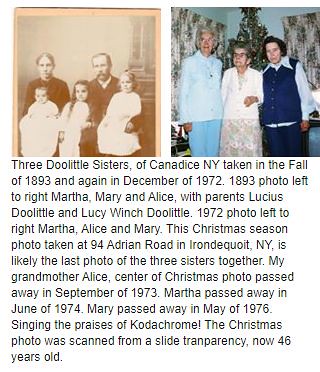The image consists of two photographs side by side, with the older photo in black and white located in the upper left-hand corner. This 1893 photograph, taken in Candace, New York, features a couple and their three children, all dressed in 1800s-style clothing. Standing left to right in this photo are the Doolittle sisters: Martha, Mary, and Alice, along with their parents Lucius Doolittle and Lucy Winch Doolittle. The adjacent, more recent photograph from December 1972, shows the now elderly Doolittle sisters—Martha, Alice, and Mary—posing in front of a Christmas tree at 94 Adrian Road in Irondequoit, New York. The scene is set against pale blue walls with visible curtains. This Christmas season photo, likely the last of the three sisters together, is noted for being scanned from a Kodachrome slide, preserving its vivid colors. Beneath the images, a caption offers additional context, including the passage dates of the sisters: Alice (center in the Christmas photo) passed away in September 1973, Martha in June 1974, and Mary in May 1976.